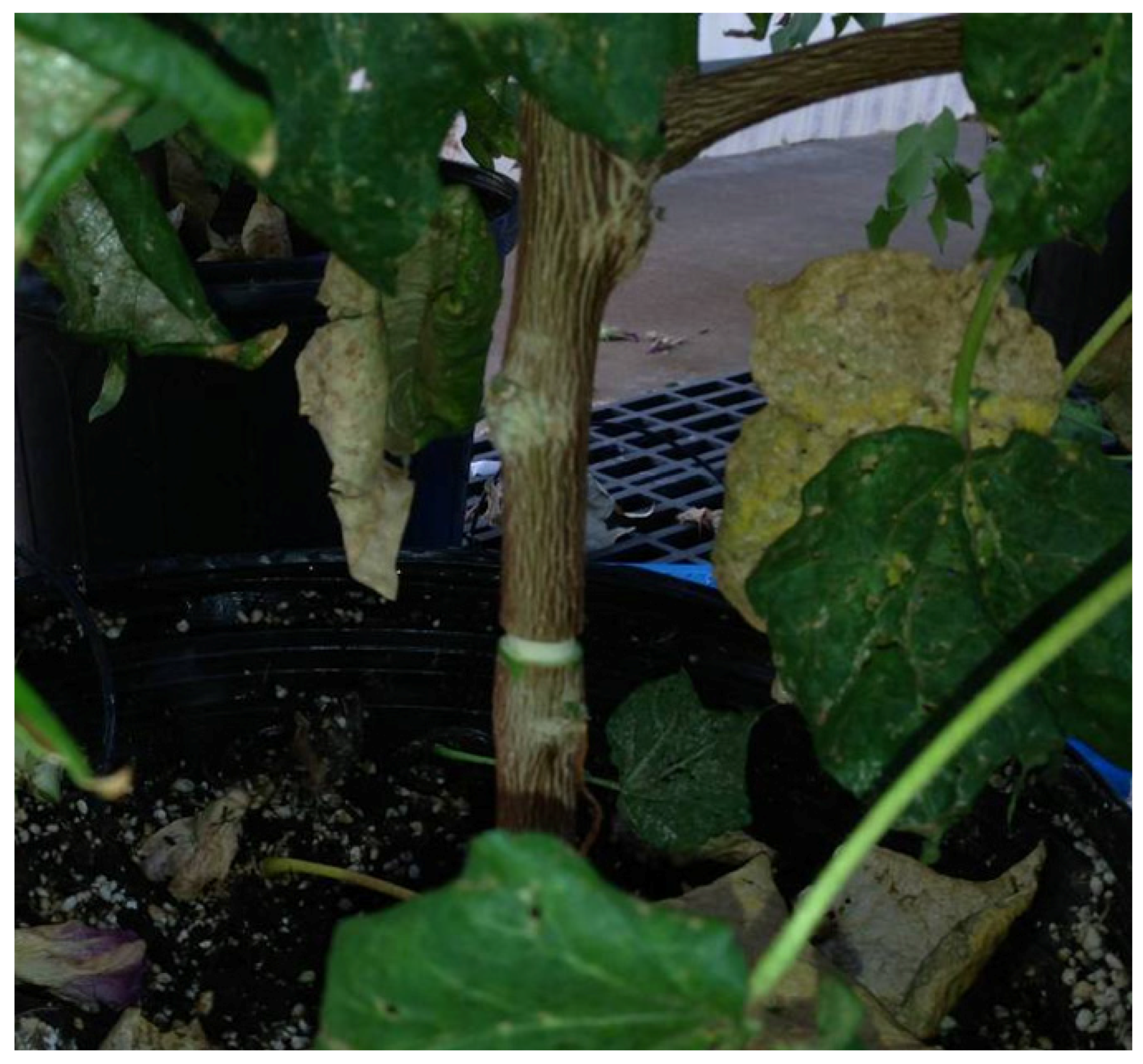This color photograph captures a close-up, zoomed-in view of a medium to large-sized potted plant, sitting inside a black pot. It features thick, hand-sized, brown stems or trunks, some of which have incisions resembling cuts that remove parts of the bark. The vibrant yet troubled plant is surrounded by dark green, lush leaves, although some leaves appear yellowing, brown, and unhealthy-looking. These leaves cascade from the branches and some are even scattered dry and crispy in the potting soil below. In the backdrop, through the foliage, a grate can be seen along with a glimpse of a concrete ground and possibly a black rubber mat, akin to those found in garden centers or greenhouses, suggesting an outdoor enclosed environment. This detailed depiction delivers an intimate glance as if one is peering closely from behind into someone's personal garden area.